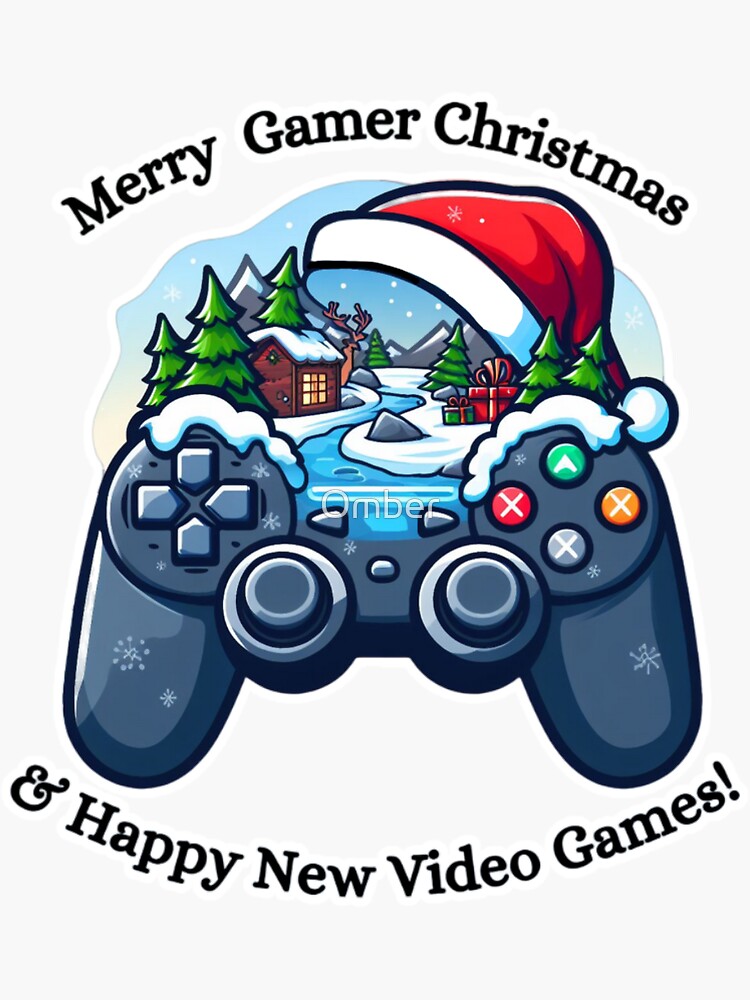The image features a detailed, cartoony illustration with a thick black outline. At the top, black serif text reads "Merry Gamer Christmas" and curves along the top edge, while opposite it, downward-curving text reads "& Happy New Video Games." Central to the image is a game controller, primarily inspired by the PlayStation design, with a bluish-gray hue and colorful buttons, where the top green button has a white triangle and the others have white X's. 

Above the controller, integrated into the illustration, a snowy landscape unfolds. Snow piles up on the top left and right sides of the controller, morphing the middle part into a light blue river with white snow snaking around it. The river leads into a picturesque scene with a brown log cabin topped with snow, surrounded by green pine trees. To the right of the river, red and green wrapped presents sit beneath more pine trees. A moose stands in the distance, with a mountain range in the background. Overhead, a giant red Santa hat with a white band and pom-pom adds a festive touch, set against a light blue sky dotted with white snowflakes. The entire composition resembles a greeting card, exuding a cheerful and whimsical holiday spirit.